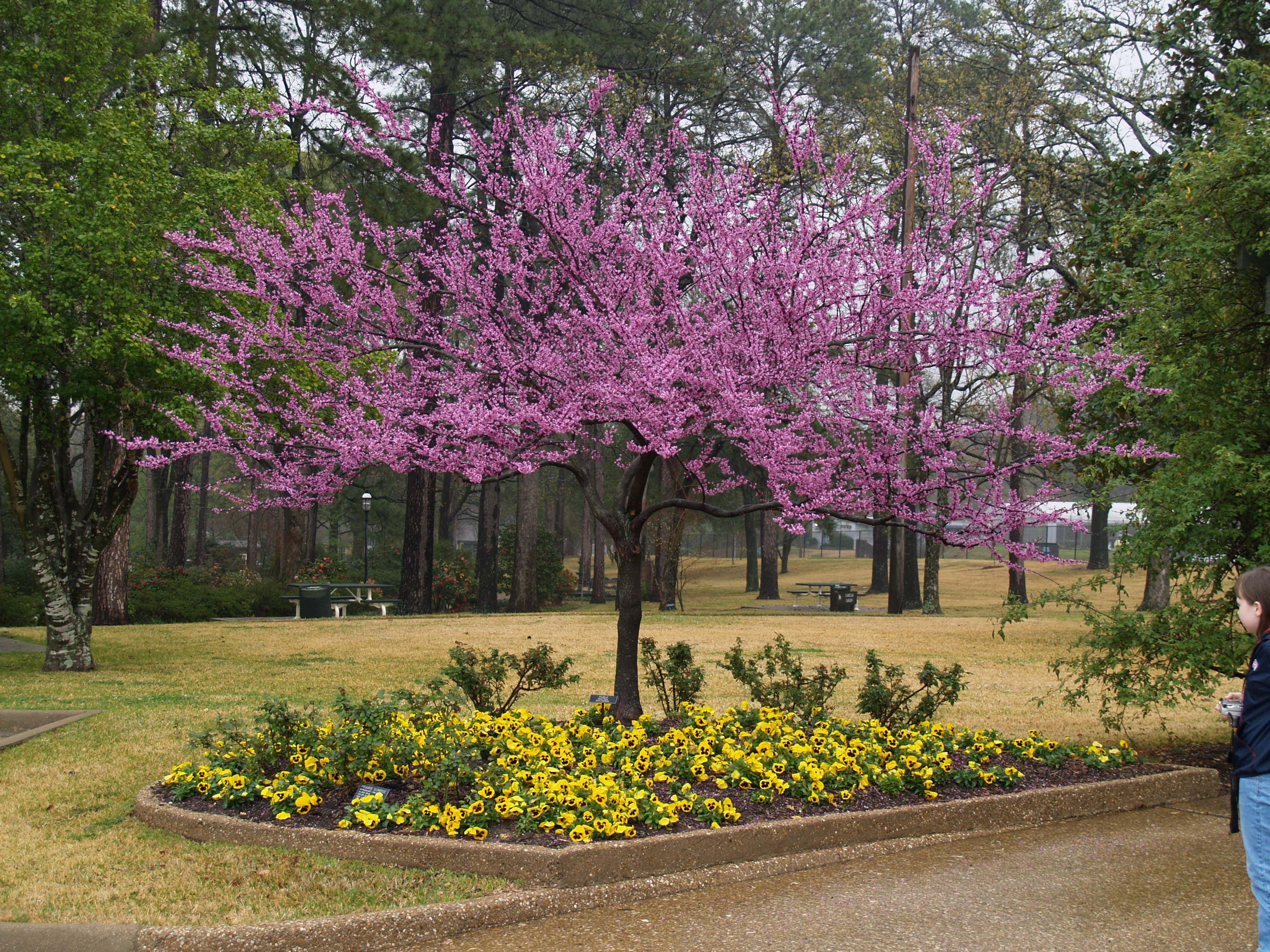The photograph, taken outdoors during the daytime, presents a scenic depiction of a park. The setting features a large, flat field punctuated by many tall trees, and various park amenities like picnic tables and benches are visible in the distance. The image, seemingly captured just after a rain shower, shows a soaking wet concrete road in the foreground, which has a distinctive brown hue due to the rain.

Central to the image is a small, landscaped area bordered by a brownish concrete perimeter. Within this area, the ground is covered with brown wood chips and dotted with small yellow flowers that have dark centers. Amidst the flowers are a few green bushes, adding to the lushness. Rising from this landscaped patch is a medium-sized tree, characterized by a thin trunk and long branches adorned with vibrant pink flowers, which appear almost purplish against the backdrop of the moist environment.

In the bottom right-hand corner of the photograph, partially cropped out, is a child or young adult. This individual is wearing a dark blue shirt and light blue pants, and they are turned in profile, gazing at the tree. The overall scene is framed by the seasonal park landscape, where patches of tan and green grass indicate the fall season.